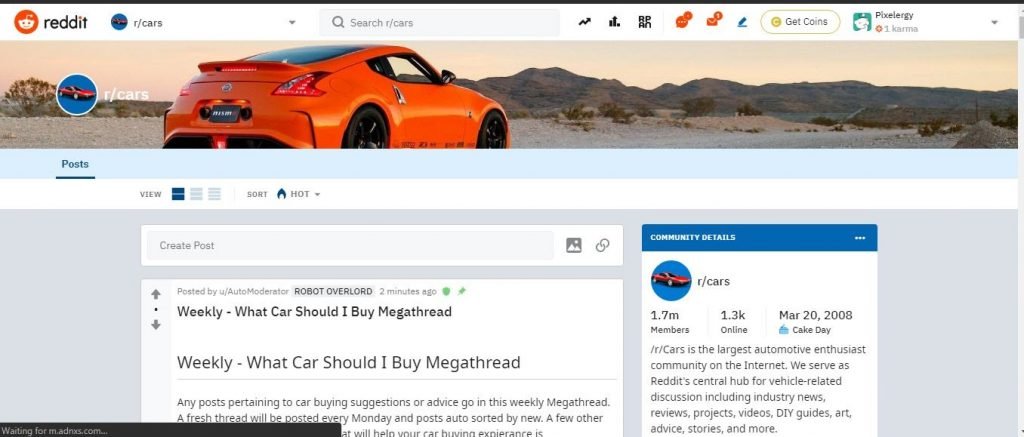The image depicts a detailed Reddit webpage, specifically the r/cars subreddit. In the upper left corner, the familiar Reddit logo featuring an orange alien head is visibly prominent. Next to the logo, the subreddit title "r/cars" is displayed, indicating the page's automotive theme. A search box is positioned to the right, allowing users to navigate Reddit's vast content. At the top of the screen, several user interface elements are visible, including icons for mail, the option to get Reddit coins, and the user profile icon for "Pixel Energy," who has accumulated one karma point.

Below the header, a banner image showcases an orange Nissan 350Z with a mountainous backdrop, reinforcing the subreddit’s automotive focus. Beneath this image lies the main post section, beginning with a pinned entry titled "Weekly 'What Car Should I Buy?' Megathread," which invites users to post their car-buying questions and seek advice.

To the right of the posts, the community details section highlights key statistics: the subreddit boasts 1.7 million members, with 1,300 currently online, and was established on March 20, 2008. The description underlines r/cars as the largest automotive enthusiast community on the internet, serving as Reddit's central hub for vehicle-related discussions, including industry news, reviews, project videos, DIY guides, art, advice, stories, and more.

The overall layout and content affirm that the image is a snapshot of a Reddit page dedicated to car enthusiasts, offering a vibrant community for engaging and informative vehicle-related discussions.